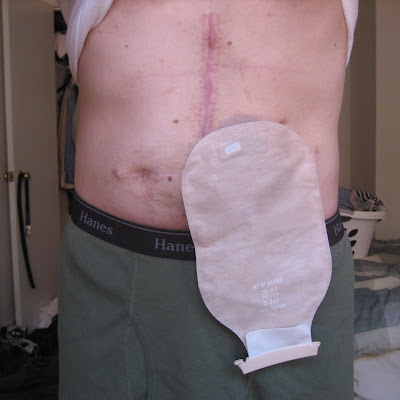The image features a person, presumably male, standing in the center of a room, with their entire body almost filling the frame. The individual is lifting a white t-shirt to expose the abdomen area, revealing a fresh, vertical surgical scar extending from the midsection of the chest down towards the navel. A drainage or surgical bag is attached to the right of the scar, partially covering the lower section of the incision. To the left of the scar, there is an indentation, likely related to the surgical procedure. The person is wearing green Hanes boxer briefs with a black waistband. The room around them includes a door on the left side with a belt hanging on the doorknob, and on the right side, a bed with a blue and white blanket. Atop the bed is a white laundry hamper containing some clothes, and a curtain hangs above the basket.